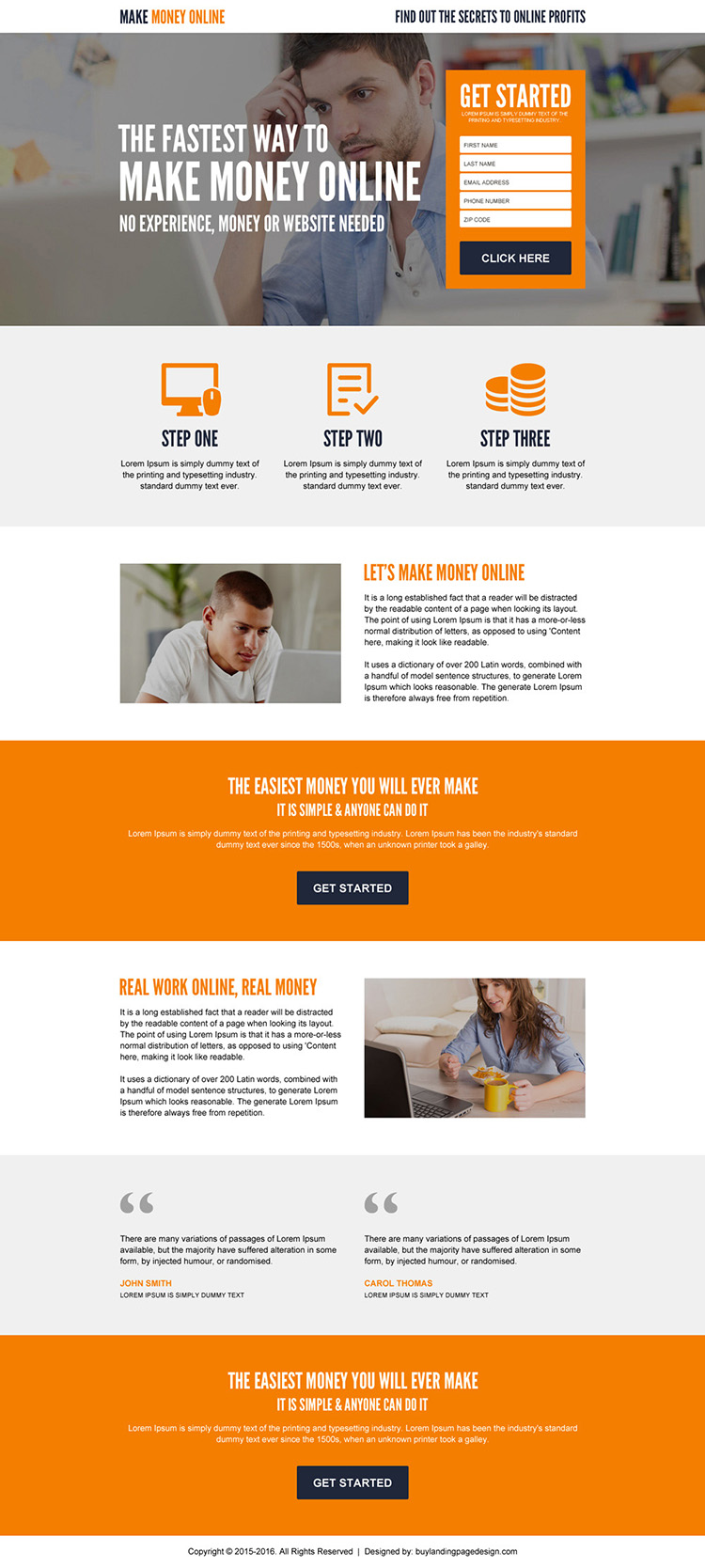The image depicts a website designed to promote earning money online. At the top, there is a banner featuring a man with his hand to his head, seemingly deep in thought while gazing at a computer screen. The heading reads "Make Money Online" and is paired with a subtitle that says, "Find out the secrets to online profits." Beneath this, a bold statement proclaims, "The fastest way to make money online."

Below the introductory text, there is a "Get Started" form where users can fill out their information, followed by a prominent "Click Here" button to proceed. Directly underneath this form, there are labeled steps titled "Step One, Step Two, Step Three," guiding users through the process.

Further down the page, there is another image of a man looking intently at a computer screen, alongside the phrase "Let's Make Money Online." Accompanying this section is an orange box declaring, "The easiest money you will ever make. It is simple and anyone can do it," along with another clickable "Get Started" link.

The bottom part of the webpage emphasizes legitimacy and ease with the tagline, "Real work online, real money." An additional orange box reiterates the message about making money and provides further instructions on how to get started.

Overall, the website appears to be a comprehensive guide inviting users to learn and engage in online money-making activities.